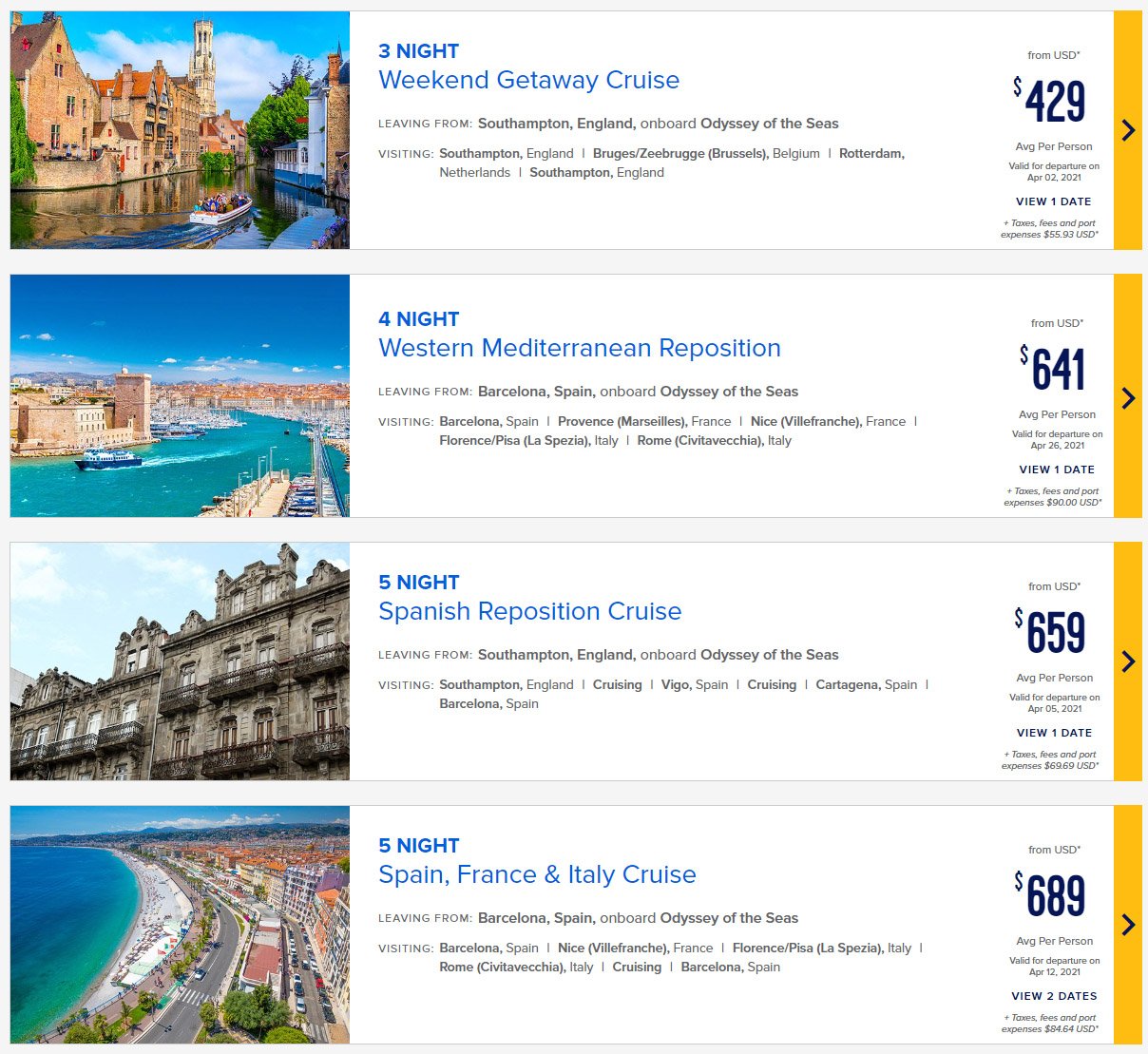This screenshot from a travel booking website displays four enticing cruise options, complete with vibrant photographs of the featured destinations. 

1. **Three-Night Weekend Getaway Cruise**: Priced at $429, this option showcases a picturesque European setting with charming buildings bordering a tranquil canal. Notable is a yellow bar indicator on the right side.

2. **Four-Night Western Mediterranean Reposition Cruise**: At $641, this itinerary features an aerial view reminiscent of the canals of Venice, highlighting a large boat cruising through teal-colored waters.

3. **Five-Night Spanish Reposition Cruise**: For $659, travelers can explore a destination highlighted by a striking old stone building, flaunting a gray Baroque facade distinct of historical architecture.

4. **Spain, France, and Italy Cruise**: This $689 cruise presents an aerial shot of a beachfront lined with apartments, high-rises, a coastal road, and a slim stretch of sandy beach, offering a glimpse into vibrant coastal life.

Additional details reveal departure points from South Africa and England on board the Odyssey of the Seas, including a comprehensive list of visiting locations for each cruise.